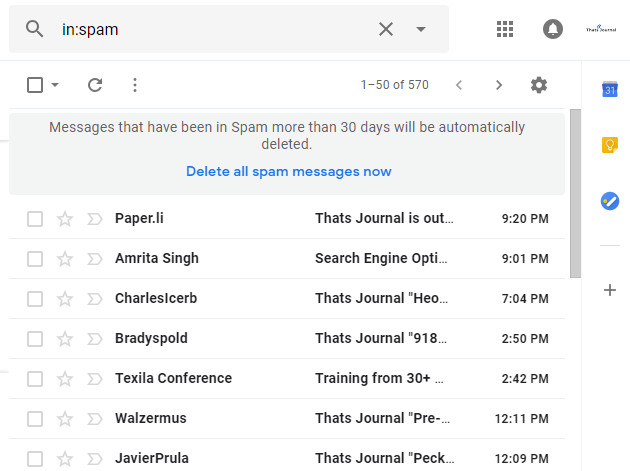The image displays the spam folder of a Gmail inbox. At the top, a clear label indicates that the user is viewing the spam folder, with options to search within the folder or cancel the search positioned nearby. On the right side of the interface, there are nine square icons representing various options and settings for the account, including alarm settings and account management. A checkbox allows users to select multiple emails at once, either to perform bulk actions or to deselect them. Currently, the inbox shows emails 1 to 50 out of a total of 570 spam messages.

To the right, several icons offer various functionalities, though their specific purposes are unclear, potentially signifying dates or other actions. The folder contains seven highlighted spam emails. Each email entry presents a checkbox on the left for selection, a star icon likely for marking important messages, and a right-facing arrow which may be used either to open or respond to an email.

The emails are from seven distinct senders, with subjects hinting at the nature of the messages. Topics range from journal publications and search engine optimization offers to training opportunities, each flagged as potential spam. Although each email shows the time it was received, specific dates are not provided.